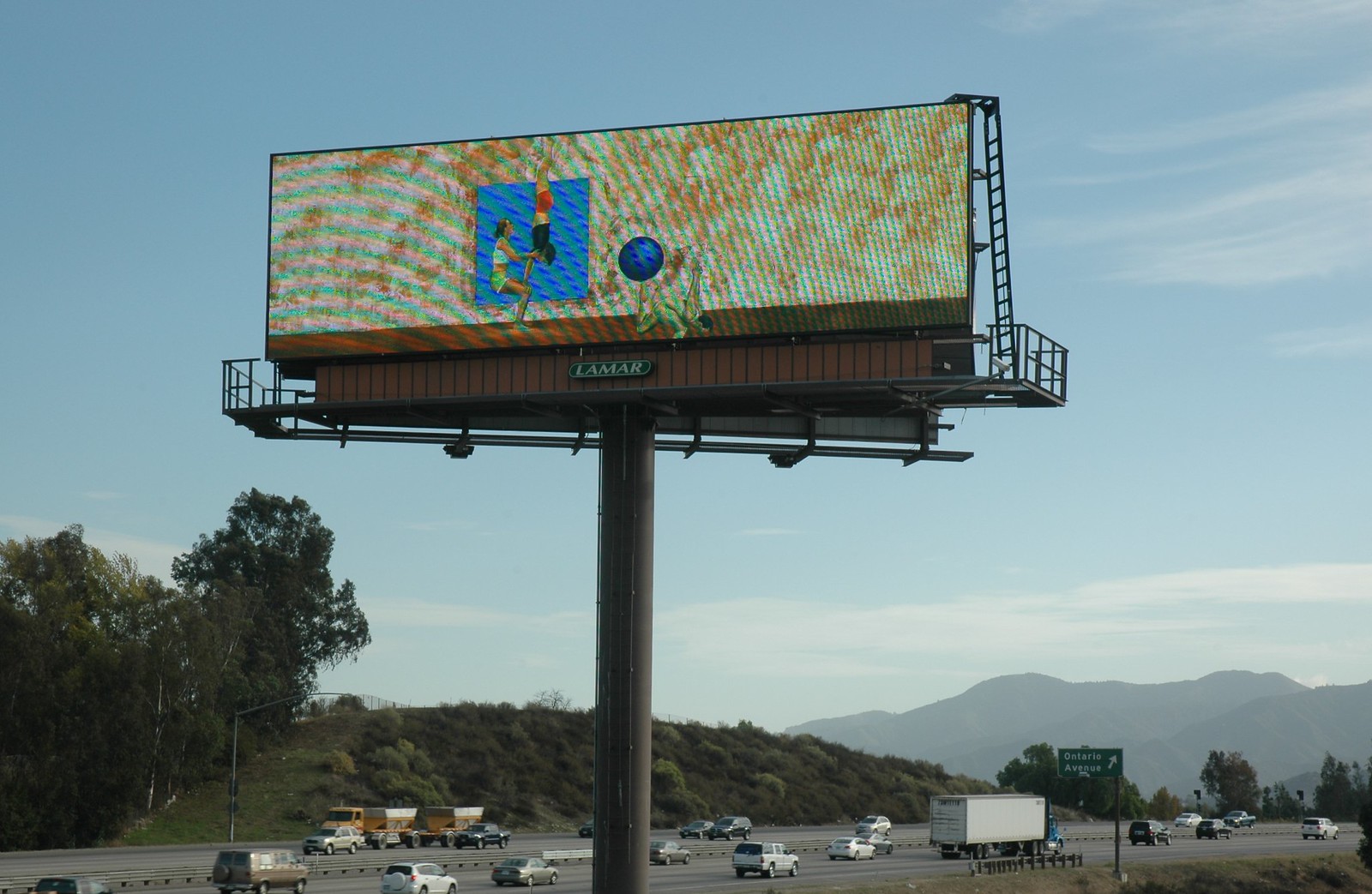In this vibrant color photograph, we are presented with a distant view of an interstate highway, prominently featuring four lanes, two in each direction, visible at the bottom of the image. A green exit sign occupies the bottom-right corner, providing a hint of color coordination with the cool hues of the landscape. Dominating the photo, the expansive blue sky stretches across, partly adorned with scattered clouds. The bottom-right corner also reveals a distant mountain range, faintly blue and serene. Centrally positioned at the top of the photograph, a large billboard draws the eye. The billboard's beige background hosts a small, turquoise square image depicting three individuals engaged in gymnastics, adding an element of dynamic activity to the otherwise tranquil scenery.